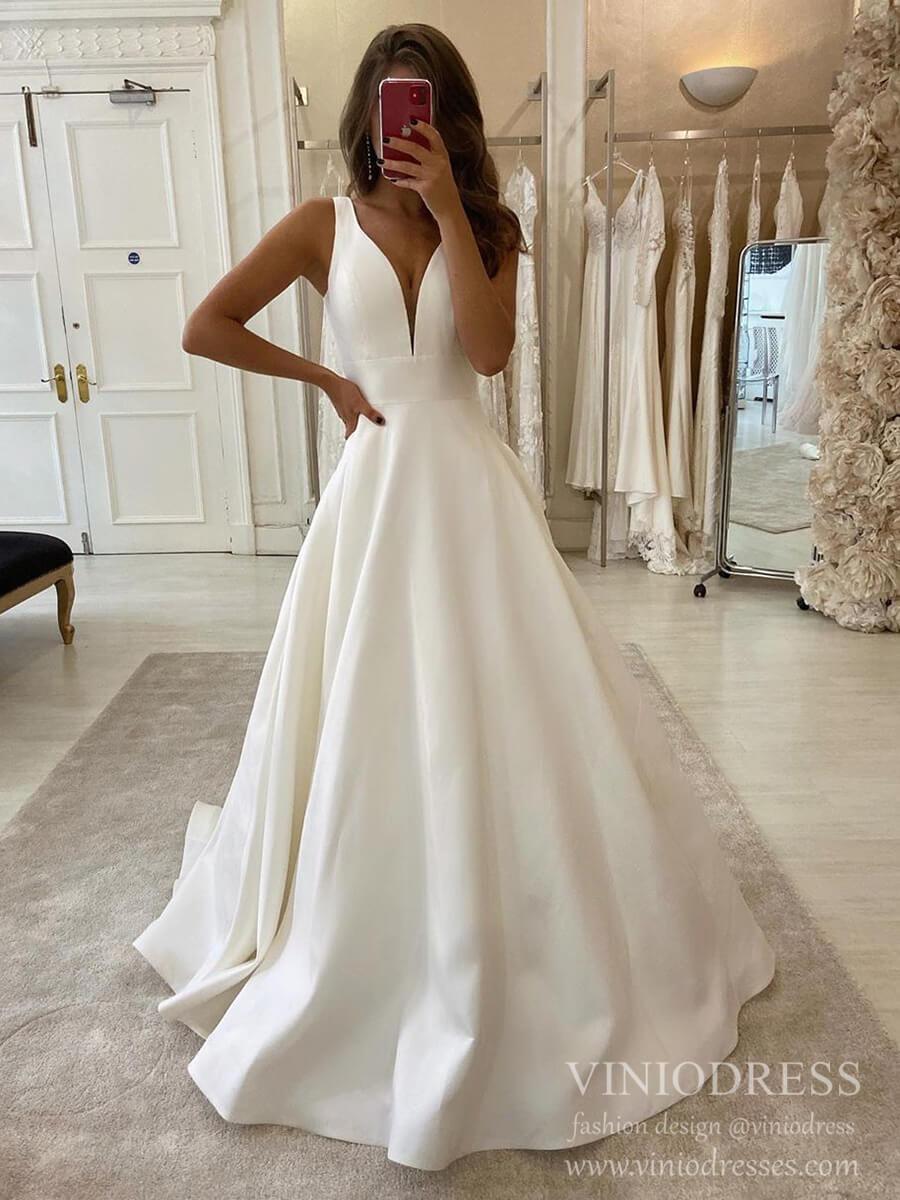In the center of the image stands a woman with tan skin and brown hair styled neatly, trying on a long, flowing wedding dress that is low-cut in the front and sleeveless. The dress is simple and elegant, lacking any lace or jewels. She is positioned on a grayish carpet in a bridal selection room characterized by its off-white and cream decor. The woman holds up a red-backed iPhone in front of her face, capturing a mirror selfie. Behind her, against a tan-colored wall, hang several wedding dresses on metal rods. An ornate white double door with gold handles is visible on the left-hand side, adorned with an intricate outer border. A tall, stand-up silver mirror stands in the right-hand corner, next to a pillar covered in artificial white flowers. An ornate footed bench adds to the room's opulent feel. On the lower right corner of the image is a watermark in white lettering that reads, "Vino Dress, Fashion Design at Vino Dress, www.vinodresses.com."